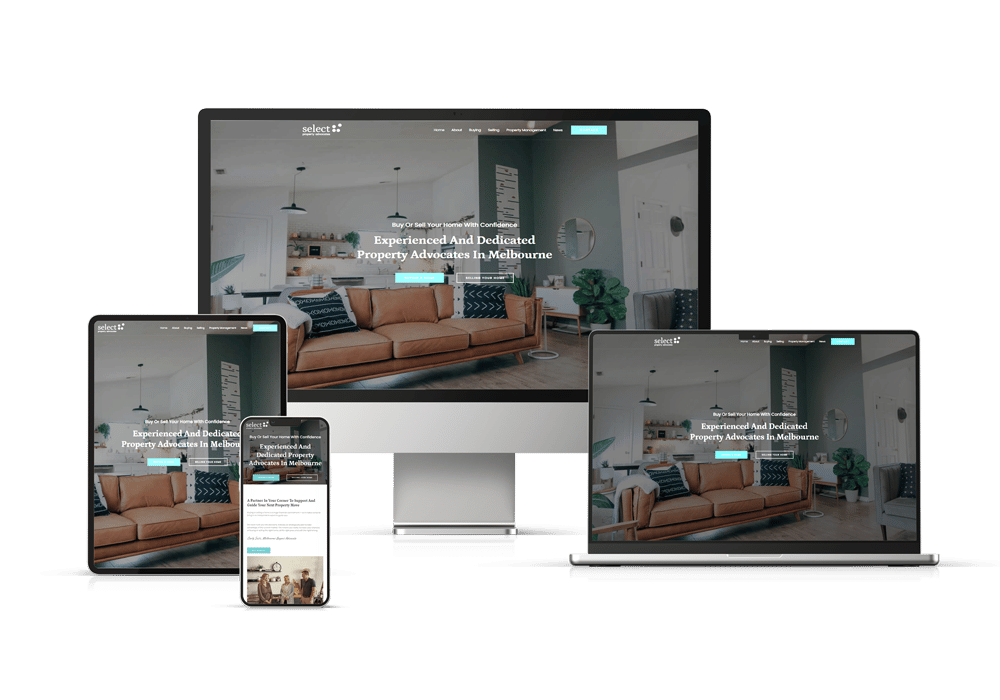The image displays the interface of a property advocacy website across four different devices: a desktop monitor, a laptop, a tablet, and a mobile phone. Centered on these screens is the same advertisement, showcasing the website's responsive design capability. The primary focus of the website, visible on the desktop monitor, is on property advocacy services in Melbourne. The scene in the background of the advertisement is a stylish living room with white walls accented by gray, complemented by modern drop lights and a tan couch adorned with black and white throw pillows. The prominent headline reads "Experienced and Dedicated Property Advocates in Melbourne," with two call-to-action buttons below—a light green button with white text and a transparent button with white text. The top menu on the desktop display features six navigation options and a light green button, though the exact labels are not legible. This multi-device display effectively communicates how the website maintains its visual and functional integrity across various screen sizes.